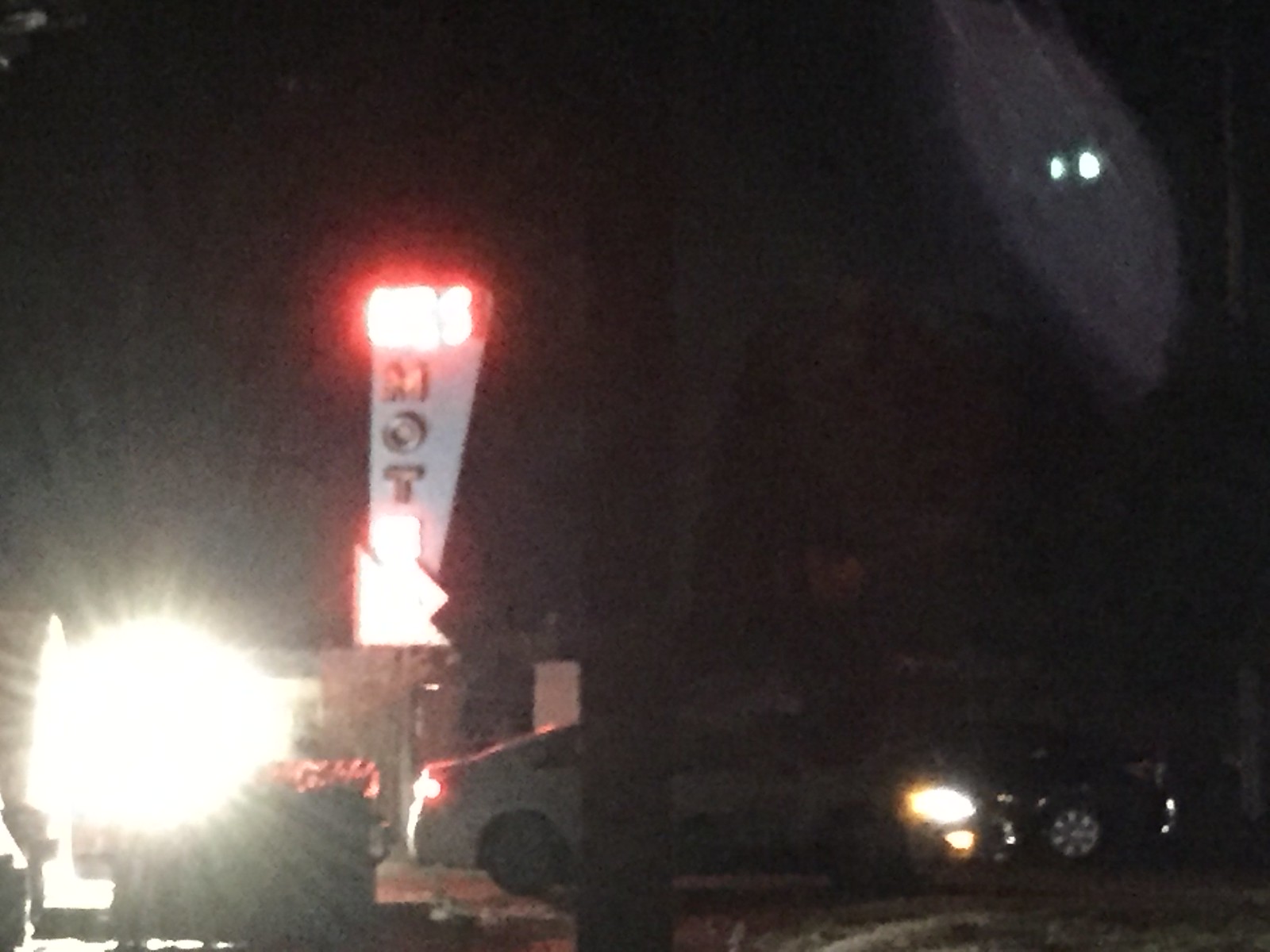On a stark black background, a captivating composition emerges. At the bottom left, a brilliant white light radiates intensely. Above this light, a prominent sign captures attention with its vivid red hue and bright illumination, bearing the inscription "MOT." Below, a car travels from left to right, its white headlights piercing the darkness while its red taillights trail behind. The scene is accentuated by another bright light situated at the top right, casting a luminous glare that extends across the top and bottom right sections of the image. Throughout the center remains a deep black expanse, punctuated sporadically by extending white lights and diffuse glare. Subtle out-of-focus artifacts encircle the edges, adding a mysterious, almost ethereal quality to the overall visual narrative.